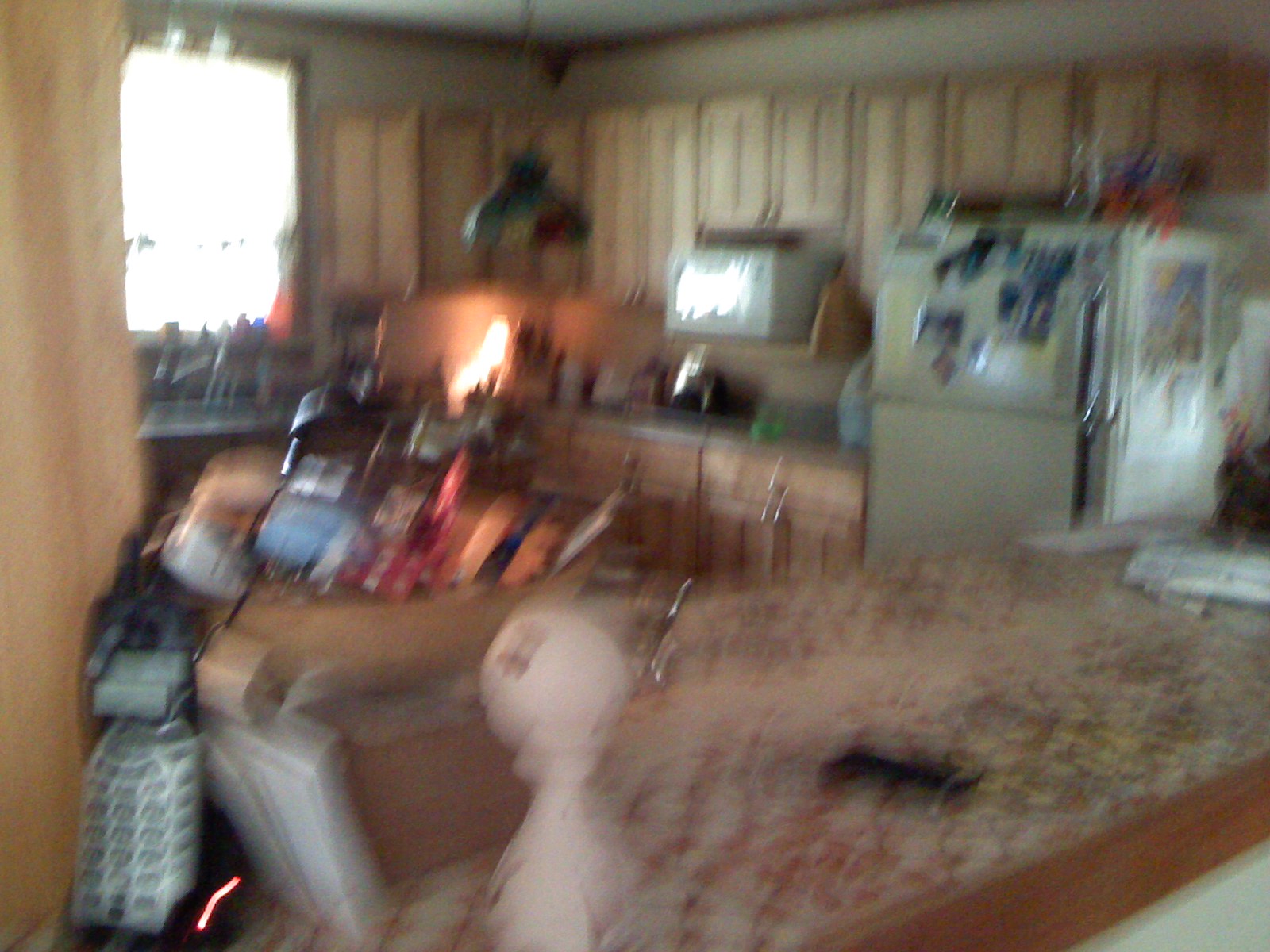This extremely blurry indoor photograph captures a cluttered and unkempt kitchen scene. On the left-hand side, there is a tan, light-stained wooden cabinet. Above it, a large, rectangular window floods the room with white sunlight. Beneath this window, a barely discernible stainless steel kitchen sink is situated. Moving upwards and to the right, the tan or off-white wall is lined with more of the same tan-colored cabinets, extending across the length of the kitchen. 

On the far right side, an older tan refrigerator, adorned with pictures, magnets, and a calendar is visible. The refrigerator's handles transition from silver to a dark wood finish. Central to the image, a grimy, worn-out kitchen island with neglected white and brown tile work and visible drag marks occupies much of the space. It appears cluttered with assorted junk. There is also mention of a countertop separating the room, potentially featuring dark gray or smoke gray surface, with a toaster on it. 

The kitchen's lower half hosts matching brown wood cabinets and drawers. On the right, a white microwave is installed on a built-in shelf. An additional standout feature is a Tiffany-style lampshade hanging from the middle of the ceiling. A chain and a shade hang down, adding to the cluttered ambiance of the kitchen.